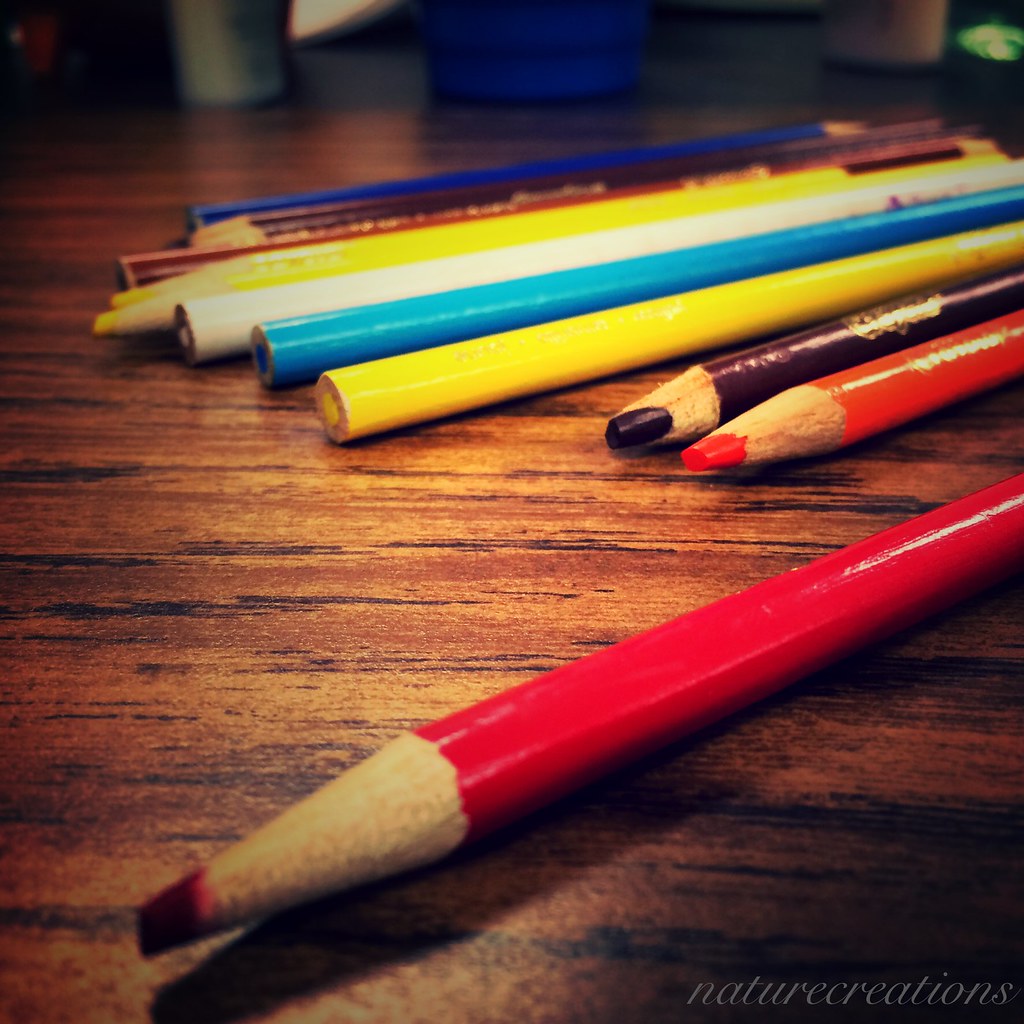This artsy indoor photograph is a close-up of colored pencils arranged on a brown formica-like wooden table with visible grain streaks. The image, titled "Nature Creations" as indicated by the computerized signature at the bottom, captures the vibrant ends and varied states of the pencils—some sharpened, some not. The colors prominently featured include red, yellow, brown, purple, blue, white, orange, potentially cobalt blue, and an additional yellow and purple. The pencils lie scattered, their ends facing in different directions, creating a dynamic composition. The background blurs into the rest of the room, focusing the viewer's attention on the richly lit pencils which stand out starkly against the table's dark wood surface.